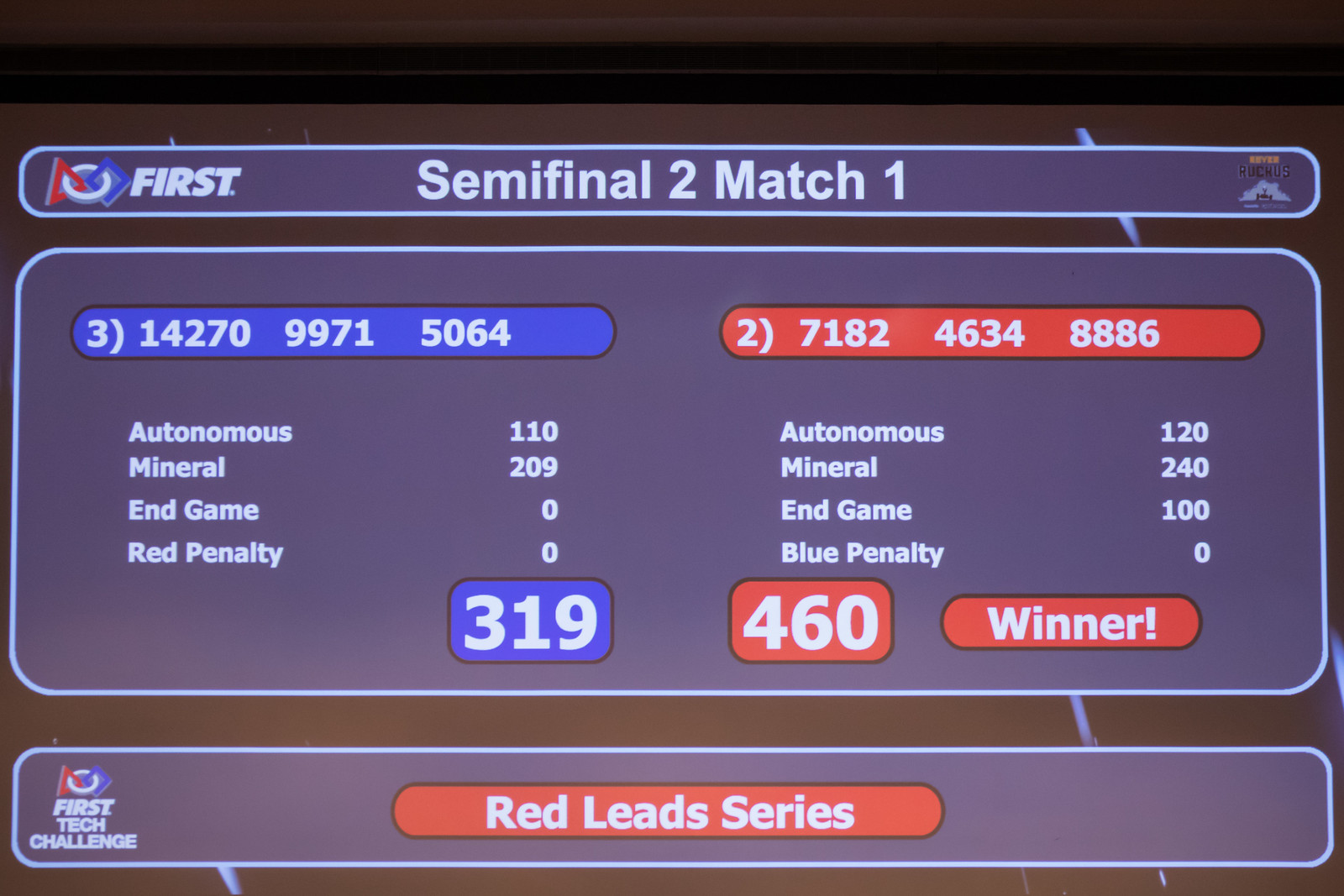The image is a digitally rendered scoreboard for a competitive event, set against a purple background. It comprises three sections in a landscape orientation.

The top section has a light blue border with a darker blue backdrop. On the left, there is an emblem, and across the top, it reads "First" in white text. Centered beneath that, it says "Semi-Final 2 Match 1," and another emblem is positioned on the right.

The central section is the widest, framed with light blue borders and a dark blue background. This section is divided into blue and red color zones. On the left, a blue bar displays the sequence "31427099715064," while the red bar on the right shows "2718246348886." Below these bars, the scores and respective phases of the competition are listed: "Autonomous," "Mineral," "End Game," and "Penalty" for both red and blue. At the bottom of this section, a blue box shows the score "319" in white text, next to a red box with the score "460" in white. Adjacent to these score boxes, there's a long red box labeled "Winner."

The bottom section is thinner and contains an emblem with the text "First Tech Challenge" underneath it. The focal point of this section is a long red box in the center that states "Red Leads Series" in white text. The prominent use of blue and red colors highlights the competitive nature of the event.